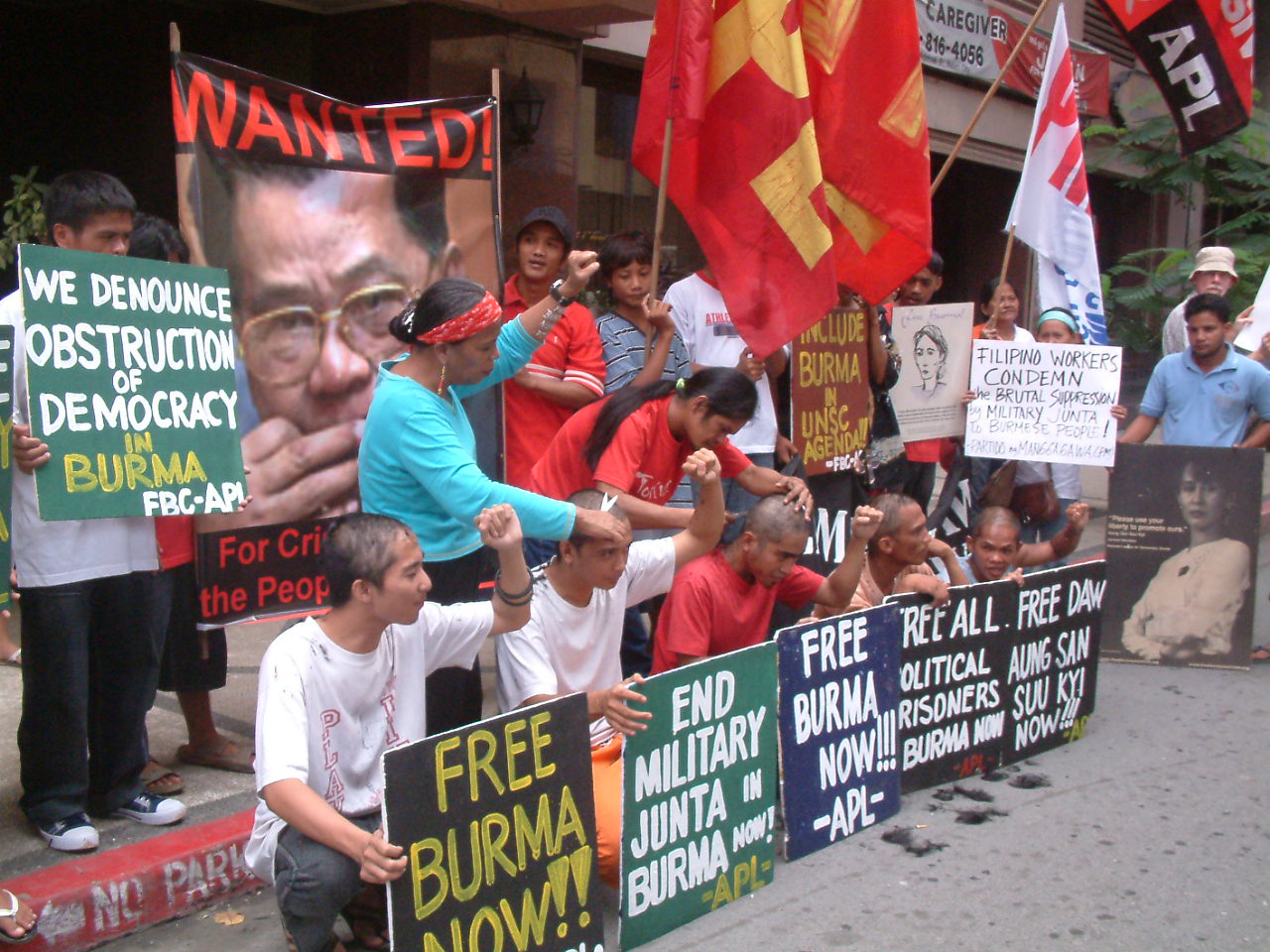In this powerful image of a protest, a group of Asian protesters is gathered along a street, kneeling in front of a sidewalk, under a bright, clear sky. They're getting their hair shaved close to the scalp by women wielding scissors, symbolizing sacrifice and solidarity. Each kneeler holds a sign, their left hands raised in defiance. The signs carry stark messages, written in various colors: "Free Burma Now", "End Military Junta in Burma Now", and "Free All Political Prisoners in Burma Now". The signs are painted in black, green, blue, and white, emphasizing a unified call for freedom and justice. Among them is a man prominently holding a sign that reads, “Free Aung San Suu Kyi Now”. Behind the kneeling men, more protesters stand, holding additional signs, one reading “We Denounce Obstruction of Democracy in Burma” and another bearing the phrase “Filipino Workers Condemn Brutal Suppression by Military Junta to Burmese People”. A striking "Wanted" poster with a man's face is prominently displayed, alongside red flags with gold lettering, contributing to the scene's intensity. They’re in front of a large building projected behind a red curb, firmly setting the event in an urban environment, making it clear that this demonstration is a highly organized call to action against the military junta in Burma.